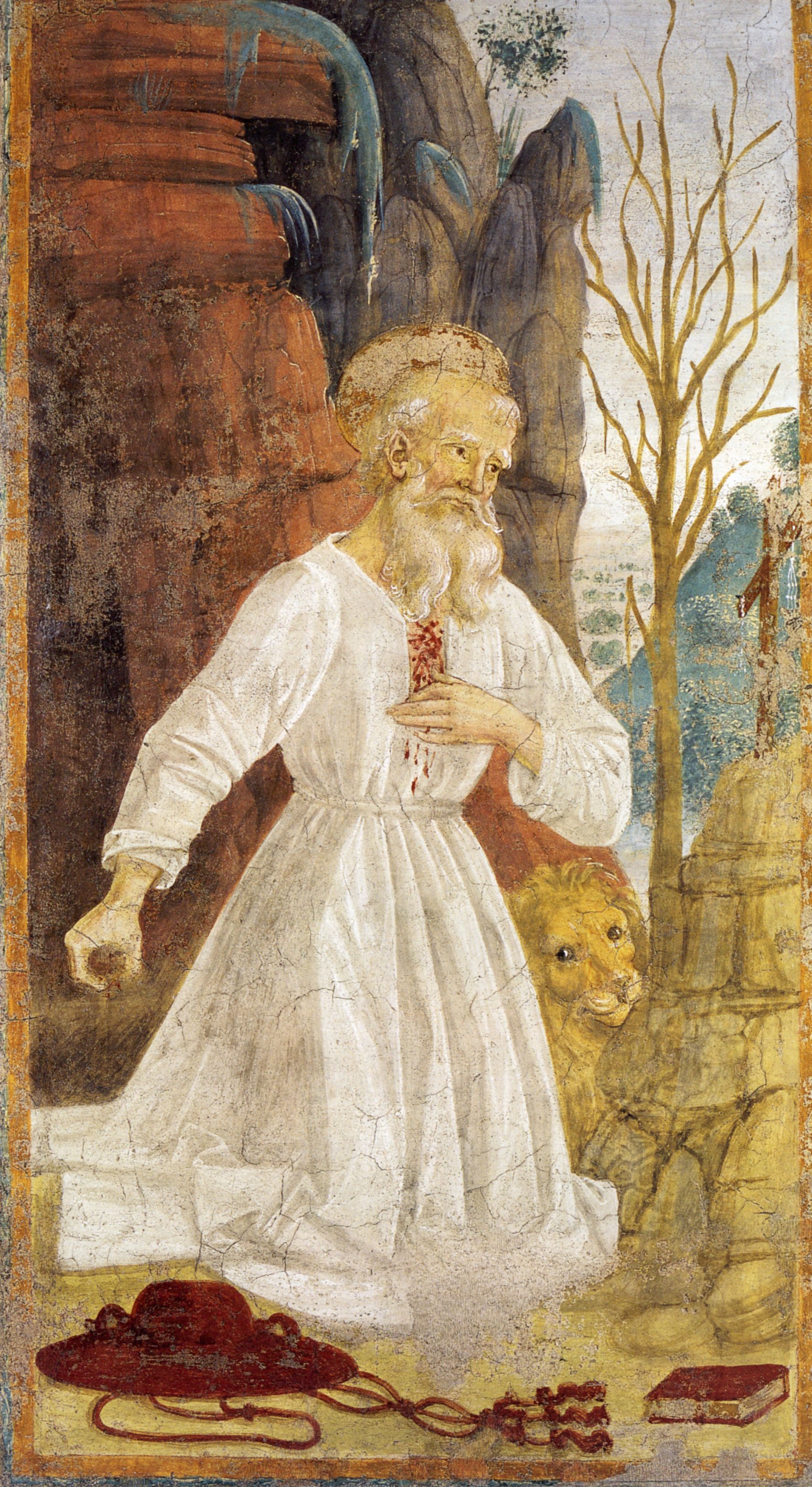The painting depicts an old man with a long white beard and mustache, dressed in a white gown, kneeling while clutching his bleeding chest. A holy, angelic halo hovers above his head, suggesting a divine or sacred figure. Behind him stands a yellow-maned lion, gazing in his direction. At the bottom of the image, a closed red book and a red hat with strings are placed on the ground. The background features a large, rocky mountain and a barren tree with no leaves, set against a clear sky. The poignant scene evokes a sense of spirituality and sacrifice.